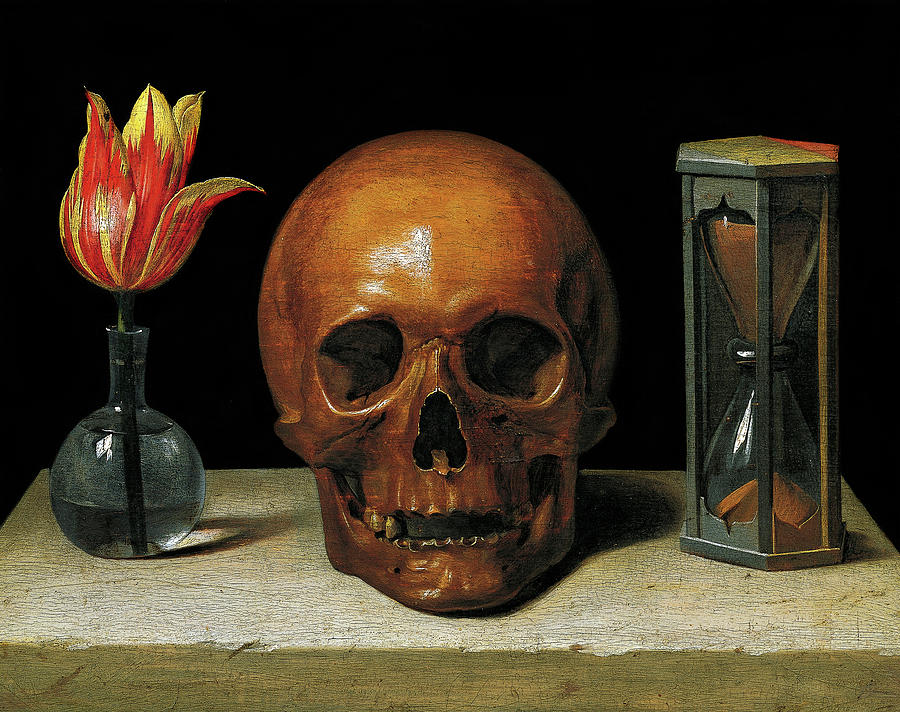This detailed handmade painting features a decaying human skull prominently centered on a weathered, tan concrete table, set against a stark black backdrop. The skull, appearing aged and damaged with only two intact teeth on its left side, is flanked by an hourglass and a vase with a flower. The hourglass, which stands to the right of the skull, is depicted with golden, black, and gray hues and shows sand trickling from the top half, still mostly full, to the bottom. To the skull's left, a bulb-shaped, clear vase is filled with water, showcasing a vibrant tulip with a green stem and striking red and yellow petals. The painting's composition is meticulously balanced, with the bottom third occupied by the concrete table and the top two-thirds enveloped in a deep, uninterrupted black background. The scene evokes a sense of transience and impermanence, with each element carefully chosen to complement the others in this classical, yet haunting still life.